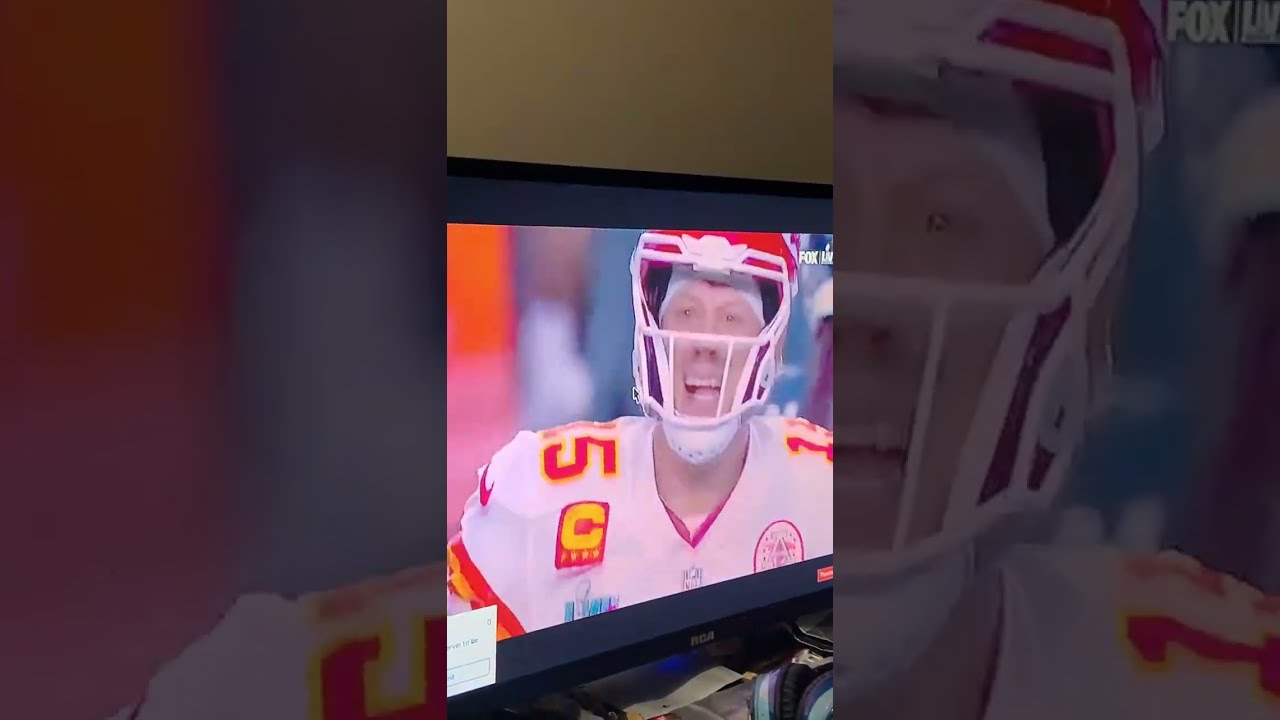The image features a photograph in a vertical strip at the center, surrounded by a blurred, zoomed-in version of the same image as the background. The central focus is a flat-screen television branded RCA, displaying a close-up of an American football player. The player, a white male, wears a red helmet and a white jersey adorned with multiple logos and the number 15 in red with yellow highlights. His mouth is open in what appears to be an expression of exhilaration or anger. The TV screen also displays the Fox News logo in the top right corner. Below the TV, various items are scattered on a table, and the background wall is dark yellow, softly illuminated. The entire scene is captured in a cell phone-style photograph, with visible aspects of a neutral-colored section of drywall above the television.